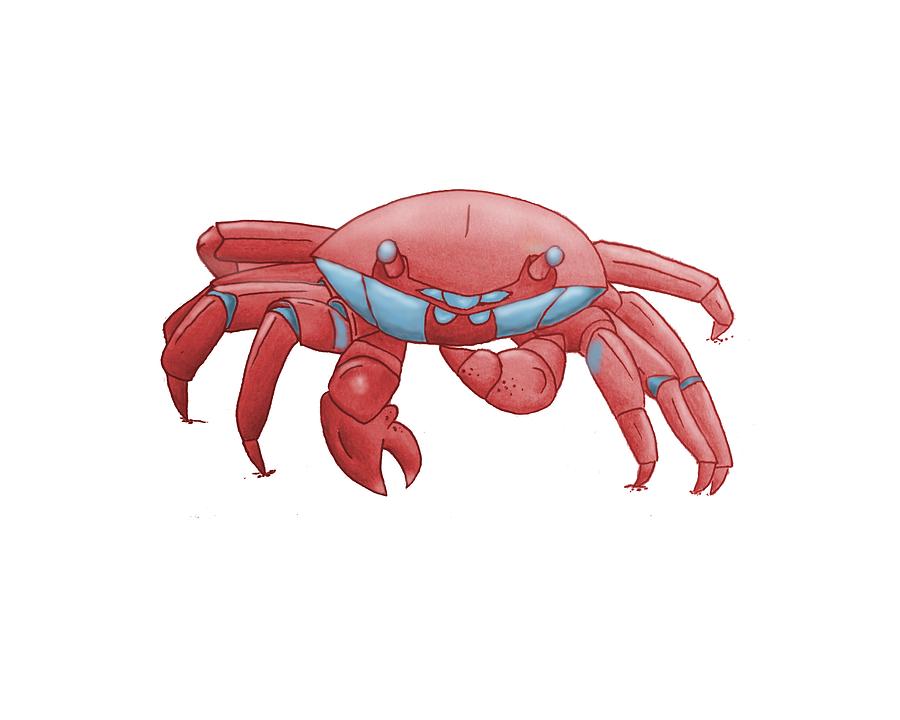This image is a detailed and vibrant color illustration of a red crab, which appears to be digitally rendered or created with watercolors and color pencils. The crab is centrally positioned and faces the viewer directly, standing on all ten legs, including its two prominent pincher claws. The claws and legs are clearly segmented, with blue joints in the middle, and the crab's small blue eyes sit on stalks at the top of its large head. The crab's underbelly and mouth also have blue accents. The illustration features a subtle shading effect, particularly on the crab's head, suggesting an overhead light source. Set against a clean, white background, the crab appears almost to float, with no other elements present to distract from its detailed depiction.